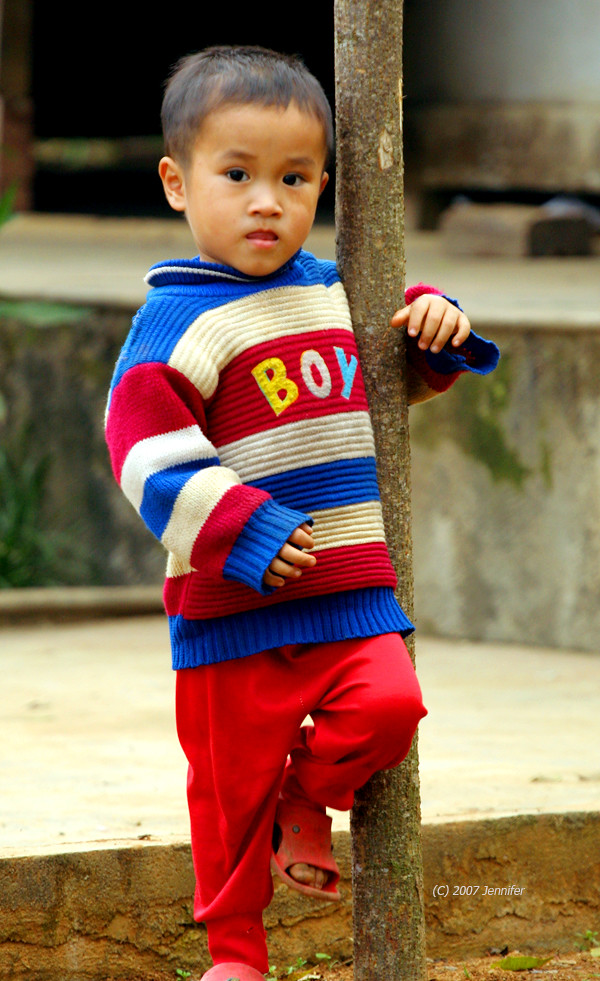A young boy of Asian descent is captured in an outdoor setting, leaning casually against a tree. His left arm wraps around the tree trunk while his left leg is lifted, knee bent. He is dressed in bright red pants and a colorful sweater featuring red, white, and blue hues with the word "BOY" prominently displayed in the center in yellow, white, and blue letters. On his feet, he sports a pair of red Crocs. His expression is neutral as he gazes off into the distance with large, contemplative brown eyes. The ground beneath him is dirt, framed by a nearby section of white concrete and an adjacent slightly elevated concrete platform.